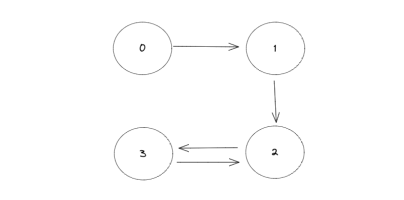The image is a computer-generated illustration appearing to depict a mathematical or scientific concept. It features four slightly elongated circles arranged in a 2x2 grid formation, resembling the corners of a square. Each circle contains a different digit, with "0" in the top-left circle, "1" in the top-right, "2" in the bottom-right, and "3" in the bottom-left, suggesting a possible sequence or relationship.

Intricately detailed arrows connect these circles, indicating directional relationships. An arrow extends from the "0" circle towards the "1" circle, oriented horizontally to the right. Between the "1" and "2" circles, another arrow points downward. Finally, two arrows connect the "2" circle with the "3" circle: one is positioned above with the arrowhead pointing left towards the "3" circle, and another below with the arrowhead pointing right towards the "2" circle. The arrows do not fully touch the circles, maintaining small gaps that vary in width.

This diagram potentially illustrates a flow or transition between states or values, possibly within a theoretical framework or model.